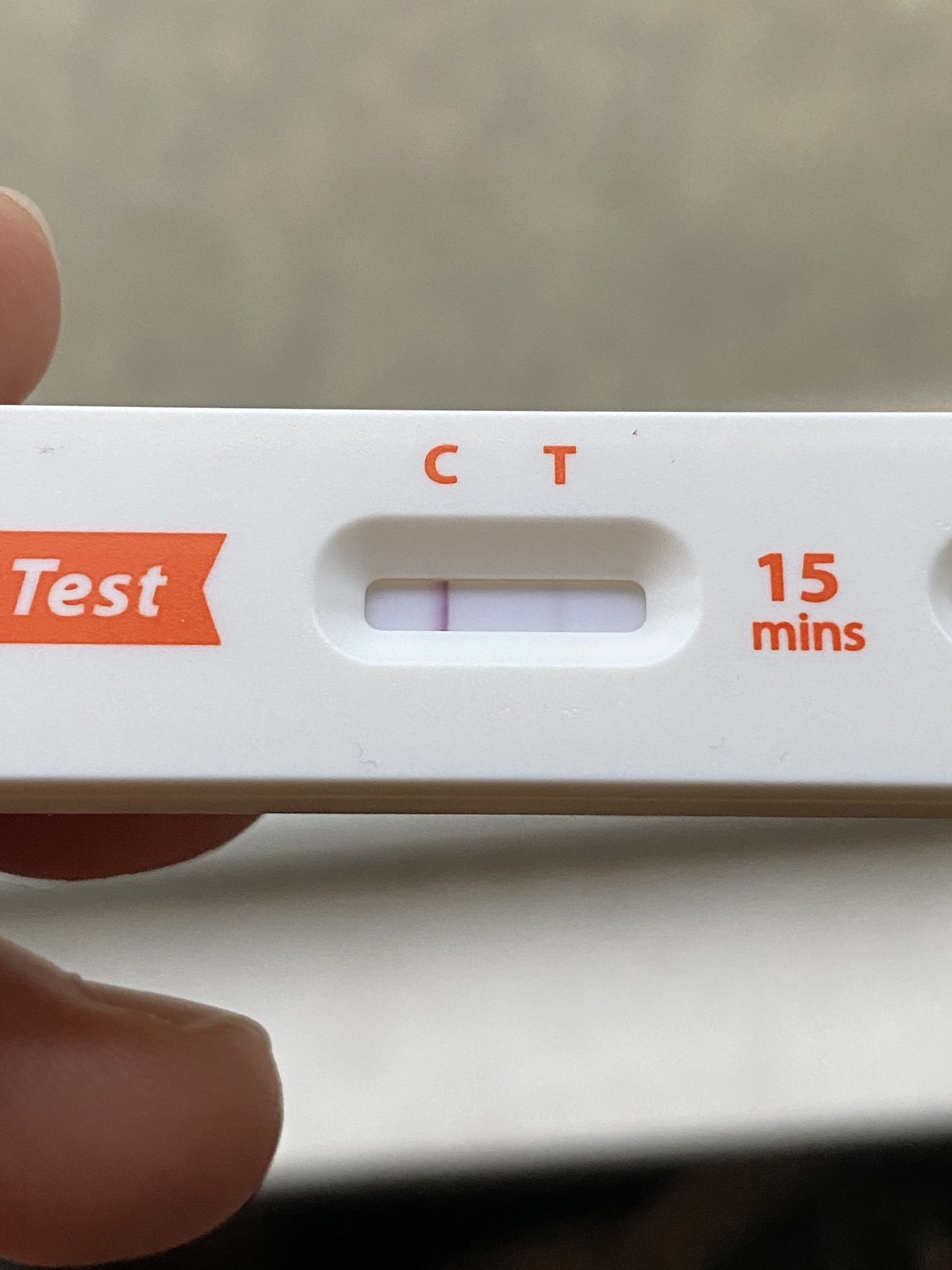This extremely close-up photograph showcases a COVID-19 rapid test. The frame is so tight that it's almost unrecognizable unless familiar with the test components. The primary focus is on the result area, where interpretations of the test's outcome seem ambiguous. In the background, the scene appears brightly illuminated, suggesting the photo might have been taken outdoors, although it could also be in a well-lit area with possible foliage or patterned wallpaper.

In the composition's lower section, there is a white surface, which could be either a piece of paper, part of the test's packaging, or a tabletop. The test device is held firmly by three fingers, which have nails approximately one-eighth inch long. The visible elements of the COVID test include its white plastic casing, an orange label that reads "test," alignments of "C" for control and "T" for test, and the "15 minutes" mark in orange.

For the results, a prominent red line is visible at the control mark "C," indicating the test's validity. However, at the "T" mark for the test result, there is a faint or emerging line, implying the results could be inconclusive or the test might not have fully developed yet. This unclear result suggests a potential repeat testing may be necessary for confirmation.

Overall, the photograph is a detailed, close-up look at the ambiguous outcome of a COVID-19 rapid test, taken against a brightly illuminated background with minimal but contextual surroundings.